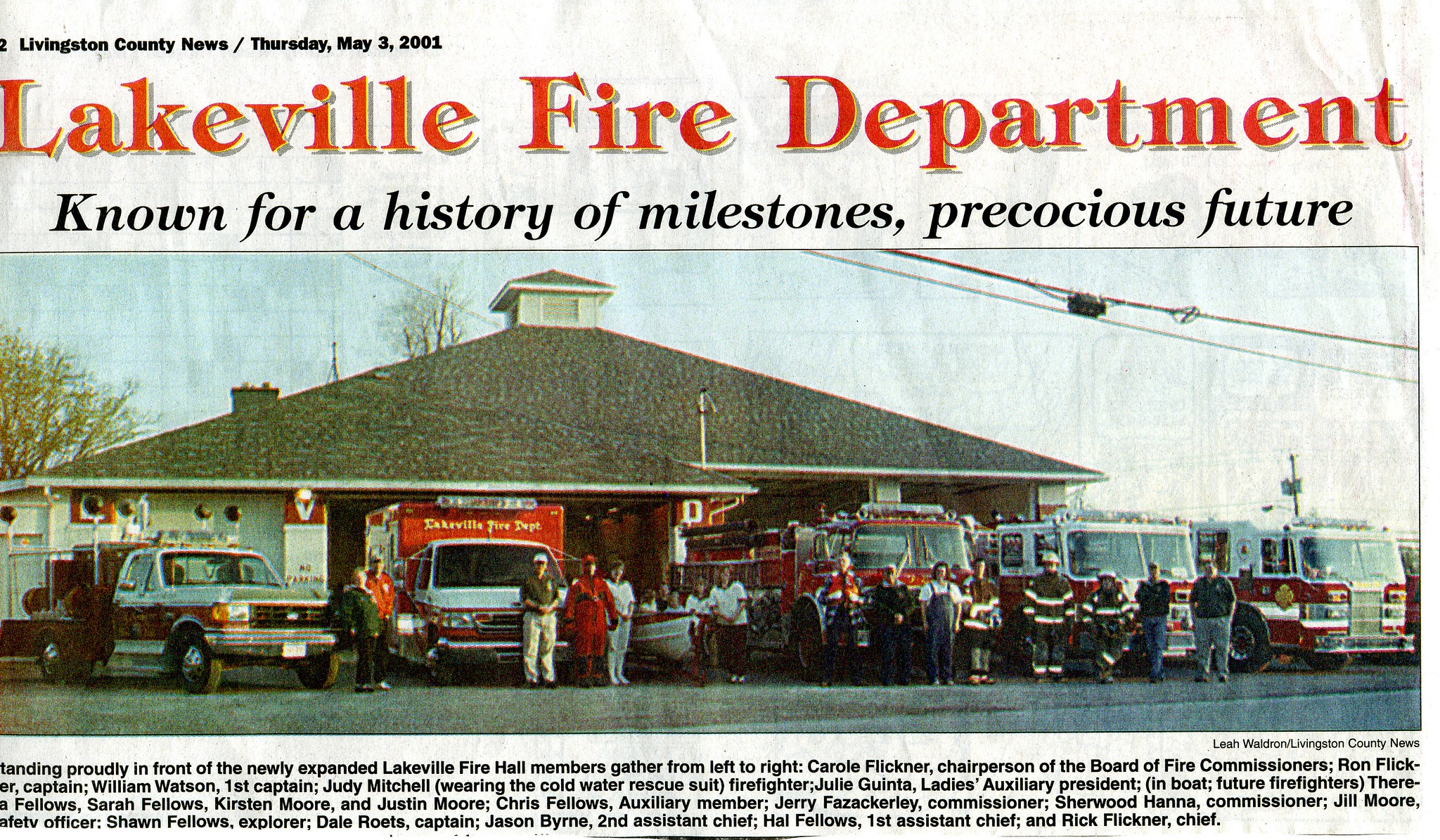The image is a color photograph from a newspaper clipping, specifically the front page of the Livingston County News dated Thursday, May 3rd, 2001. The headline, displayed in large red letters, reads "Lakeville Fire Department," and underneath, in black font, the subheading states, "Known for a history of milestones, precocious future." The wrinkled newspaper clipping showcases a picture of the newly expanded Lakeville Fire Hall. Outside the fire station, a row of various fire trucks, and possibly other vehicles, are parked. In front of these trucks, firemen and other members of the department, some in fire gear, pose proudly for the camera. The caption below the photo, partially cut off, mentions that the members are gathered "from left to right" and proceeds to list their names and roles within the fire hall.